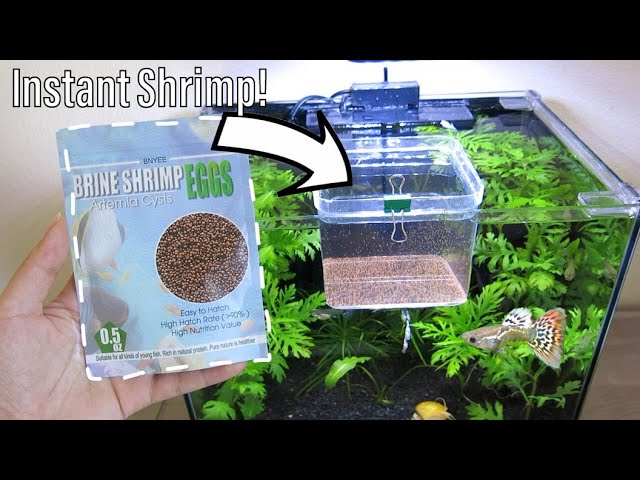The advertisement features a vibrant, eye-catching layout promoting a product prominently labeled "Instant Shrimp!" The focal point on the left side showcases a hand holding a square, blue package of "brine shrimp eggs." The package is adorned with a circular window, allowing a glimpse of the little brown granules inside. Above the window, the brand name B-N-Y-E-E is printed in black text alongside the title "Artemia cys." in green. Other notable details on the package include claims of "easy to hatch," "high hatch rate over 90%," and "high nutrition value" in black text, with additional text asserting the product's suitability for all kinds of young fish due to its rich natural protein content, though one word remains illegible.

Pointing towards the aquarium is a white arrow, bordered in black, signifying where to place the granules. The plastic square feeder, presumably bright and clear grey, is clipped to the interior of the aquarium. The aquarium itself is brimming with water and filled with fake green plants, providing a lively backdrop. Inside the tank, there are visible aquatic inhabitants: a distinct guppy with an orange tail marked by black and yellow spots on the fins and tail, a green body, and a golden snail nestled at the bottom where black pebbles lie. Another fish with a big fan tail and polka dots also swims nearby, enhancing the vivid and detailed depiction of the scene.